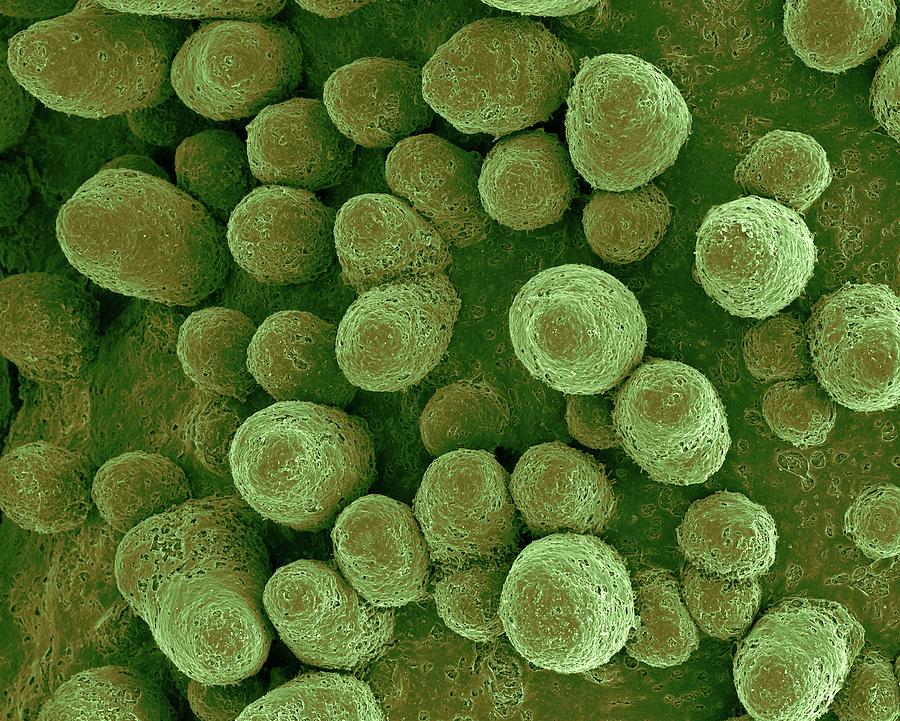The image features an enigmatic close-up that evokes a sense of natural mystery. Set within a green and brown landscape, the photograph captures an irregular pattern of cylindrical and egg-shaped objects resembling either spores, cocoons, or even rocks filtered in green hues. These objects, varying in size from tiny diamonds to quarters, are dispersed unevenly across the surface. Some are clustered in groups while others stand alone, showing a range of sizes and shapes—some wispy and string-like, others more robust and round, all with small holes throughout. The underlying surface ranges from dark grass green to light, almost whitish hues, adding to the overall sense of depth and complexity. Shadows interplay with light, creating an image both beautiful and mysterious, inviting viewers to imagine hanging it on their wall as an intriguing piece of art.